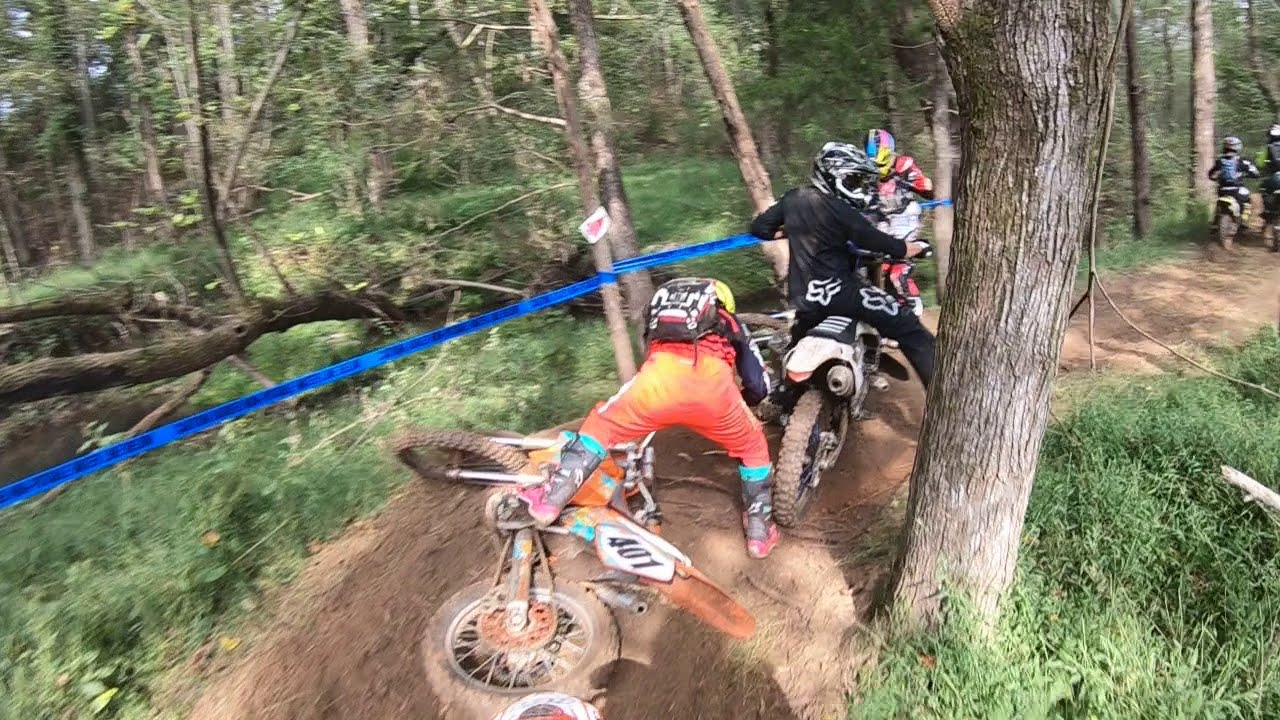The image depicts a dirt motorbikes competition set outdoors on a narrow, brown soil track that cuts through a densely forested area. The track, lined with green grass and trees, is filled with several dirt bikers, but the focus is on an incident at the center. Here, a dirt bike numbered 401, which is orange, blue, and pink with white trim, has fallen to the ground. The rider, dressed in a matching uniform with a yellow helmet and a backpack, is visibly trying to lift the motorcycle back up while on their feet. In close proximity, another rider dressed in black appears to be glancing back toward the fallen biker. Further ahead on the track, more dirt bikers are visible, continuing the race. The forested surroundings include both standing trees and some that have fallen, with a blue strip forming a boundary on the left side of the track.